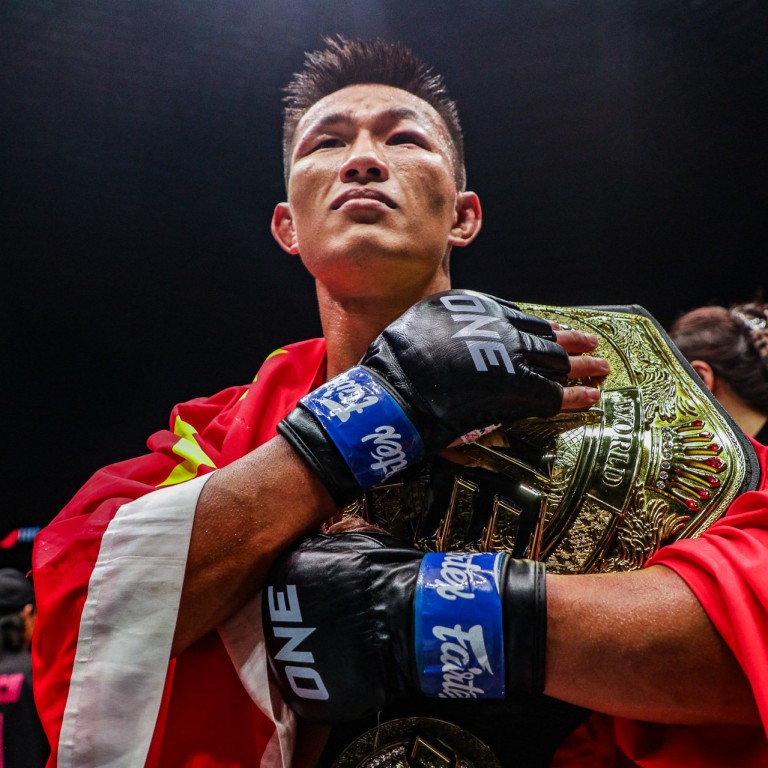The image is a close-up portrait of a Japanese fighter, identifiable by his Asian descent, darker brown skin, and short, spiky black hair. He has a slightly swollen face, particularly around the eyes, and no facial hair. He is wearing black, fingerless leather gloves with blue accents around the wrists, and the number "1" is visible across the knuckles. Draped over his shoulders and torso is a red and yellow robe with white borders on the sleeves, which might also be interpreted as a flag indicating his victory. Across his left shoulder, he proudly holds a large, ornate golden championship belt. His arms are crossed over his chest, and he gazes slightly upwards and to the left. The background is predominantly black, and there is an indistinct figure behind him, partially obscured by his shoulder and the belt. Other undefined objects are visible on the left side of the image.